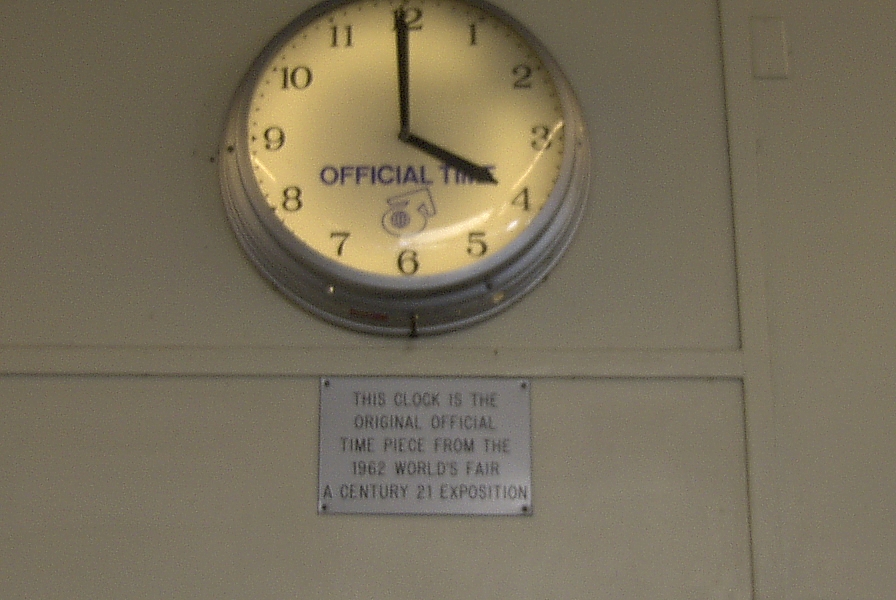In this picture, mounted on a light tan, white, or grayish wall that appears to be part of a ship's interior, is a historically significant clock. The clock's casing is a silver or gray oval, featuring a classic design reminiscent of naval timepieces. It has a white face with large, easy-to-read black numbers and black hands, indicating it is four o'clock. The clock's face is illuminated from the back, highlighting its historical significance. Below the clock, a silver placard bears the distinct message in black letters: "This clock is the original official timepiece from the 1962 World's Fair, a Century 21 Exposition," held in Seattle. The clock also has the words "Official Time" written in blue across the bottom, accompanied by a blue circle with an arrow pointing upwards towards the time. A small logo is positioned above the six on the clock face. This well-preserved artifact stands as a timeless testament to the grandeur of the 1962 World's Fair.